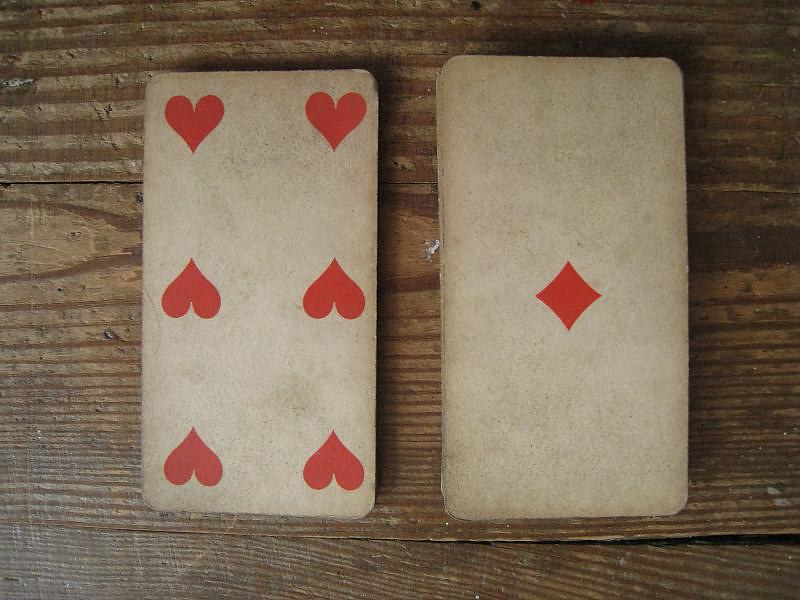A photograph of two well-worn playing cards resting on a distressed and aged wooden table, which is composed of three visibly distinct wooden boards. The table's surface is heavily scarred with scratches, giving it a timeworn appearance. On the right side of the image lies the Ace of Diamonds; on the left is the Six of Hearts. The cards show signs of age and frequent use, with evenly dispersed staining and slight fraying around the edges. The Ace of Diamonds is more stained compared to the Six of Hearts. The designs on the cards are minimalistic, featuring only the suit symbols without any numbers. The Six of Hearts displays four hearts facing downward and two facing upward, while the Ace of Diamonds showcases a single diamond at its center.